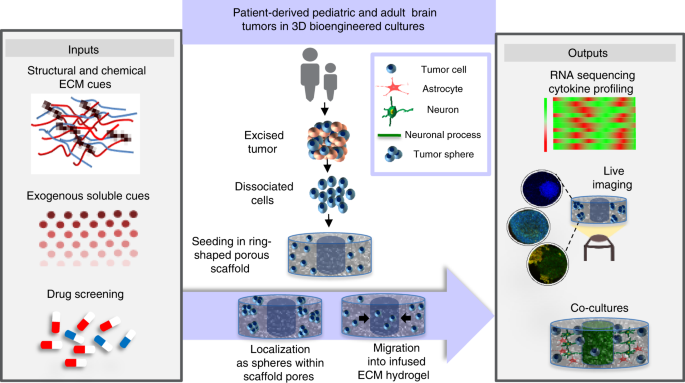This image is a detailed professional scientific diagram centered around "Patient-derived pediatric and adult brain tumors in 3D bioengineered cultures," displayed prominently on a purple backdrop. The diagram is divided into three main sections: inputs, the central experiment, and outputs. 

On the left, inside a gray box, the inputs are listed, including "structural and chemical ECM cues," illustrated with blue and red squiggly lines, "exogenous soluble cues," depicted by a gradient of colored dots transitioning from dark brown to light pink, and "drug screening," represented by red and white capsules. 

In the center, the process of the experiment is shown with various illustrations. Starting with "excised tumor" shown as blue and pink orbs, moving to "dissociated cells" depicted as blue spheres, seeding into "ring-shaped porous scaffolds" shown as cylinders filled with spheres. The process continues with localization as spheres within scaffold pores and migration into infused ECM hydrogel. There are human figures of a child and an adult at the top, alongside several cell types: tumor cell (a small blob), astrocyte (a pink star), neuron (a green object), neuronal process (a green bar), and tumor sphere (three blue orbs).

On the right, the outputs are listed in another gray box, including "RNA sequencing" with red and green striped blocks, "cytokine profiling," "live imaging" represented by globes and cylinders in various colors, and "co-cultures" depicted by a cylinder with green in the middle and red, white, and blue around it. 

The overall design integrates multicolored graphics throughout, linking textual descriptions with vivid visual representations to illustrate the complex process of studying brain tumors in engineered 3D cultures.